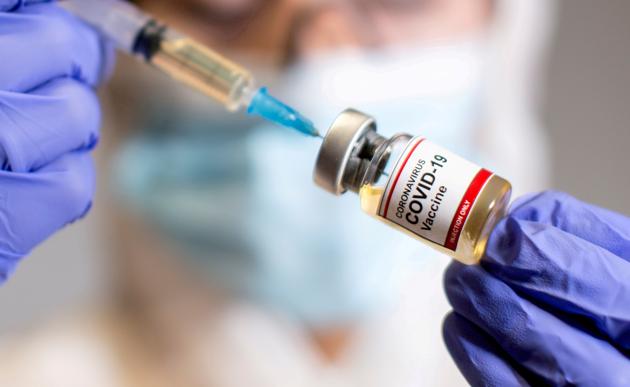In this detailed image, a medical professional is meticulously drawing up a dose of the coronavirus COVID-19 vaccine into a syringe. The focus of the photograph is on the gloved hands of the healthcare worker, who is wearing purple nitrile gloves. The syringe, featuring a yellowish-colored liquid, has a blue plastic cap at the base of the needle. The needle is inserted into a clear glass vial bearing a white label that reads "coronavirus COVID-19 vaccine" and is topped with a silver lid. The background is intentionally blurred, revealing the healthcare professional clad in a white hazmat-style suit with the hood up and a blue and white medical mask covering their face. This setup creates a sterile, safe environment for handling the vaccine. The professional's careful technique is evident as they gently pull back the stopper to draw the vaccine into the syringe, preparing it for administration.